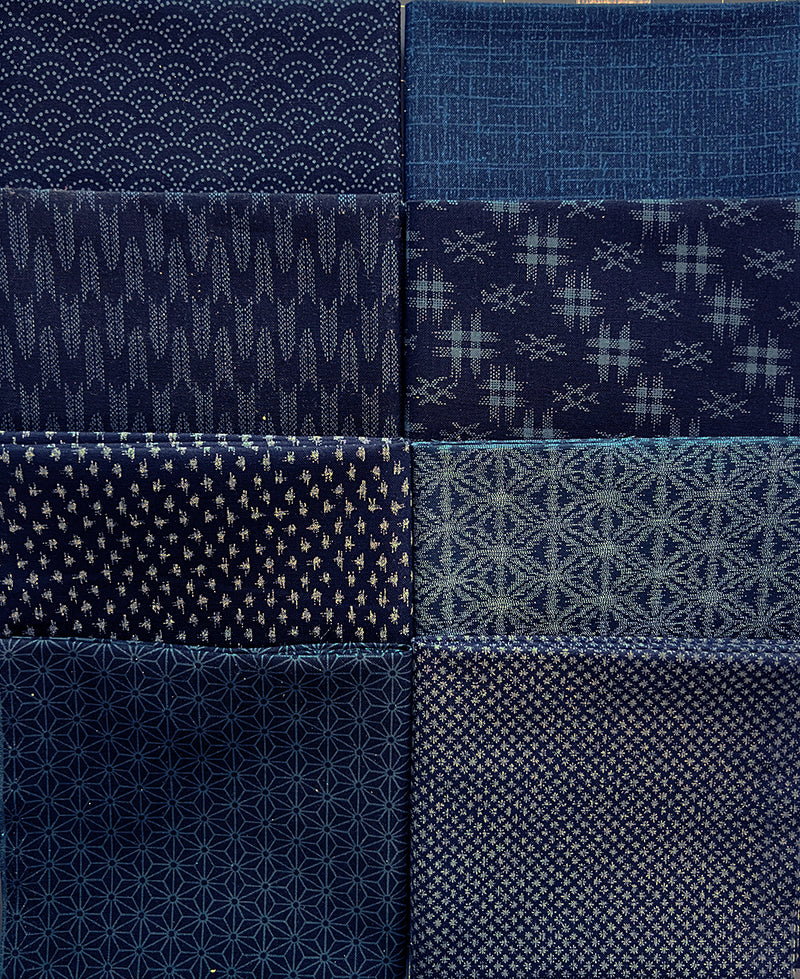The image displays eight folded sections of dark blue fabric, arranged in four rows and two columns, each showcasing distinct patterns. The top left fabric features a dark blue background adorned with repeated, scalloped white designs reminiscent of an overlapping oval sunrise. To the right, the fabric presents a lighter blue shade with thicker, randomly placed bright lines that cross-hatch horizontally and vertically, resembling TARDIS blue. Moving to the second row on the left, the pattern interweaves upward and downward arrowhead-like gray shapes against the dark blue. Adjacent to it, the right panel showcases a design marked by thin white lines creating a grid-like pattern. The third row begins with a fabric on the left that depicts small gray hashtag marks and intricate snowflake shapes, while to its right, there's a light blue fabric filled with light gray scallop designs running vertically. The bottom left shows a darker blue fabric patterned with complex, star-like geometric shapes. Finally, the bottom right fabric displays a dark blue background with vertical white designs.